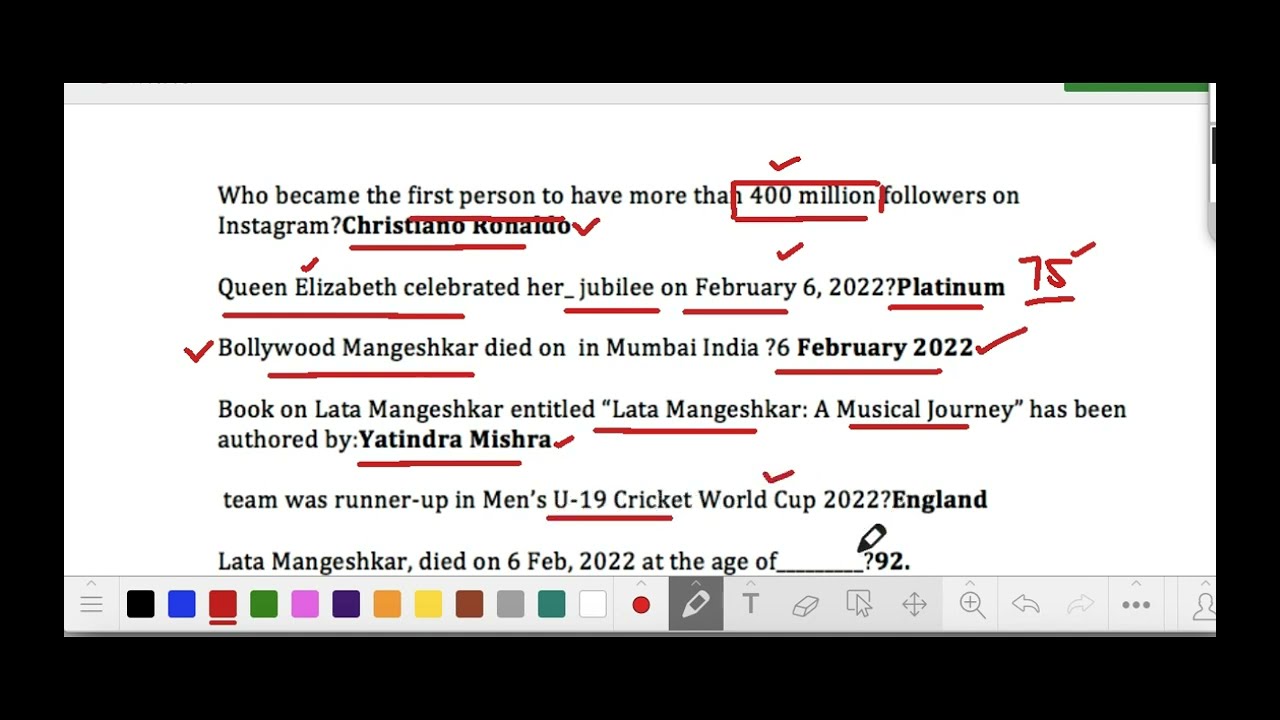The image is a screenshot from a text editor on a computer, resembling a word processing document. The central section features black text in what appears to be a Times New Roman font on a white background, which has been visibly cropped, leaving a sliver of a gray background and a hint of green. The text itself is a series of trivia questions with bolded answers and annotated in red. For example, it asks, "Who became the first person to have more than 400 million followers on Instagram?" followed by the bolded and underlined answer, "Cristiano Ronaldo." Other questions mention Queen Elizabeth's Jubilee on February 6, 2022, and Bollywood singer Lata Mangeshkar's death. Specific words and dates are underlined or highlighted in red, with annotations like checkmarks and boxes. The bottom of the screen features a menu bar with various tool icons, including color options, markers, a font eraser, and a magnification tool, indicative of the text editing environment.